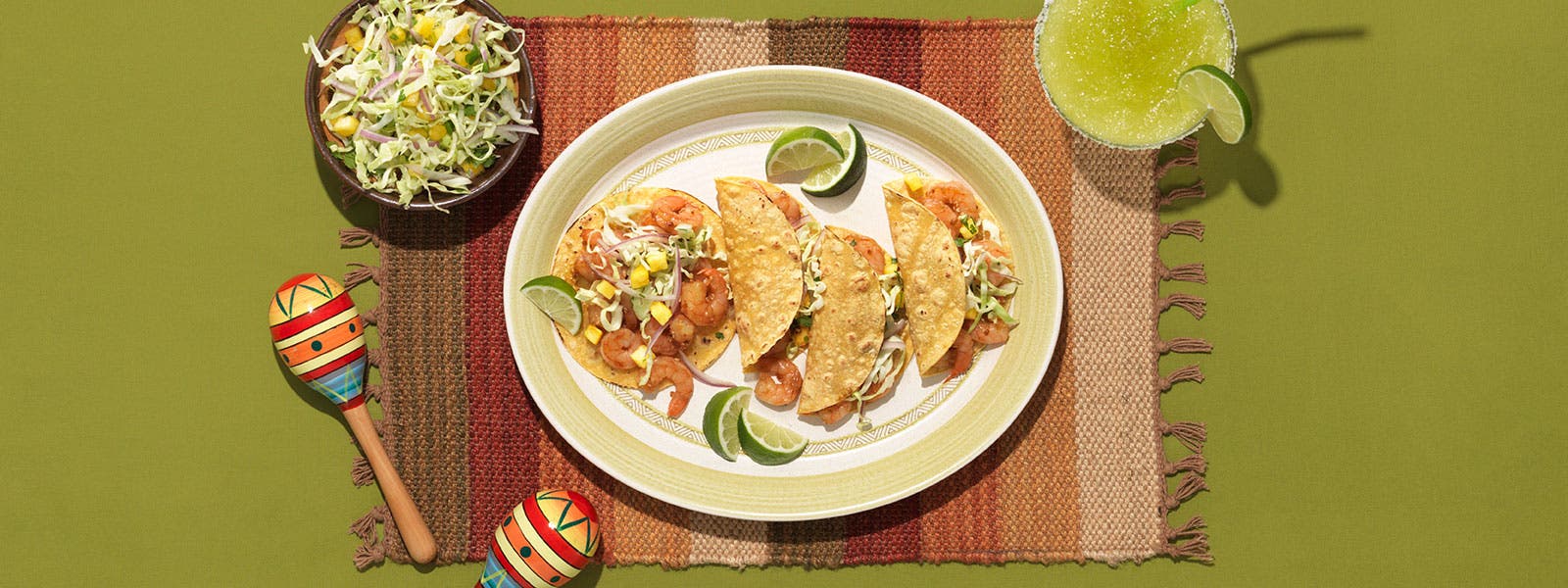On a vibrant lime green dinner table, a colorful meal is beautifully presented atop an earthy-toned placemat featuring stripes of tan, clay red, orange, apricot, and other desert hues. Central to the composition is a white oval plate with a light green-yellow edge, holding four shrimp tacos; three of the tacos are neatly rolled, while one is open to display its contents, which include shredded lettuce, red onions, and possibly mango or pineapple. Surrounding the tacos are five lime slices, invitingly positioned for squeezing. To the upper left of the plate sits a brown bowl filled with a coleslaw mix of cabbage, corn, shredded red onions, and a hint of fruit, possibly mango. In the upper right corner, a green margarita garnished with a slice of lime and a salt-encrusted rim adds a refreshing touch to the scene. Adding a festive flair, two decorative maracas with yellow, red, blue, and orange stripes rest to the lower left, enhancing the lively and inviting atmosphere of this meal.